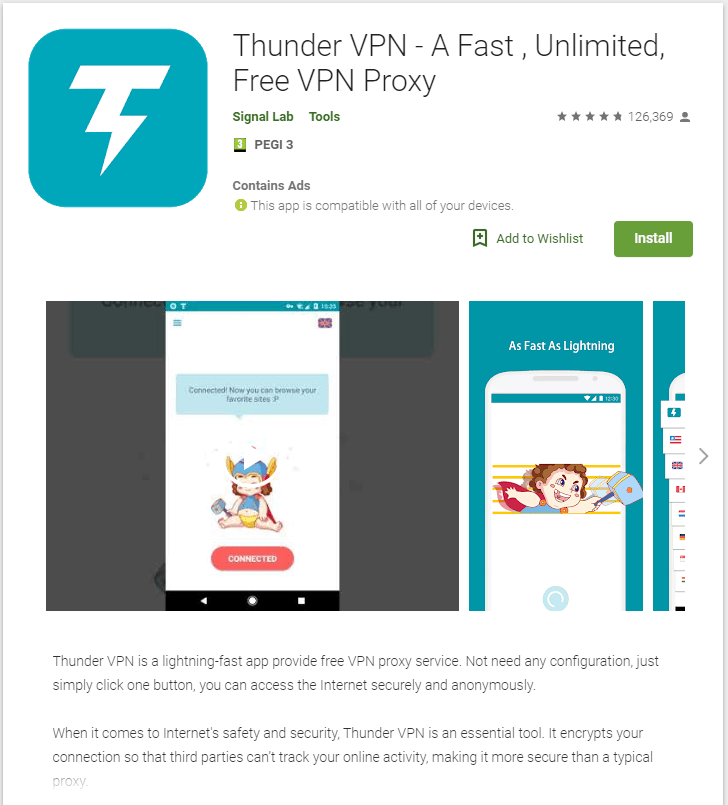**ThunderVPN - Your Ultimate Free VPN Proxy Solution**

In the image, a prominent blue square features the ThunderVPN logo, highlighting it as a "fast, unlimited, free VPN proxy." Review metrics are included, showing a 5-star rating with 126,369 users. The app is compatible with all devices, and an "Add to Wishlist" button alongside the installation prompt is visible.

A confirmation message reads: "Connected. You can now browse your favorite sites." Another section states "As fast as lightning," illustrated by a figure wielding a hammer, draped in a cape, and standing next to various flags, symbolizing global connectivity.

ThunderVPN is described as an ultra-fast application providing free VPN proxy services. It requires no configuration; a single click enables secure, anonymous internet access. Emphasizing internet safety, the service encrypts user connections, preventing third-party tracking and ensuring a security level surpassing that of standard proxies.